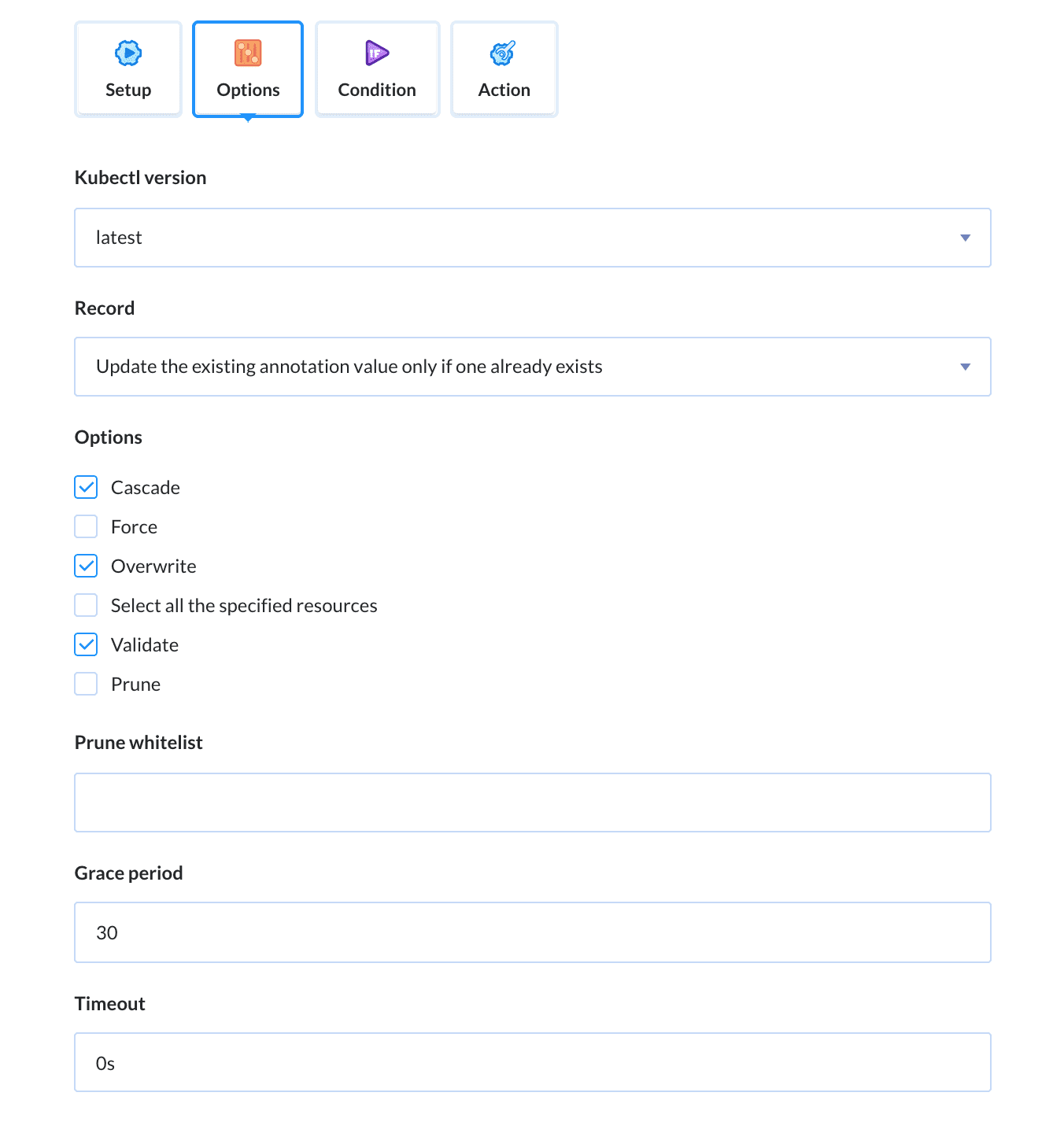A detailed screenshot of a Kubernetes workflow interface. At the top of the page, there are four small, white square icons, each representing a distinct function. The first icon is a gear, labeled as "Setup." The second icon is an orange square, labeled "Options." The third icon is a purple rectangle facing right, labeled "Condition." The fourth icon is a blue bubble, labeled "Action."

Below these icons, the text "kubectl version" is displayed, indicating the latest version of the tool. The selected record option specifies, "Update the existing annotation value only if one already exists." In the "Options" section, three choices are checked: "Cascade," "Overwrite," and "Validate." The "Prune Whitelist" field is empty, while "Grace Period" is set to 30 and "Timeout" is zero seconds.

The background of the interface is white. Additional options not checked under "Options" include "Force," "Select all the specified resources," and "Prune."